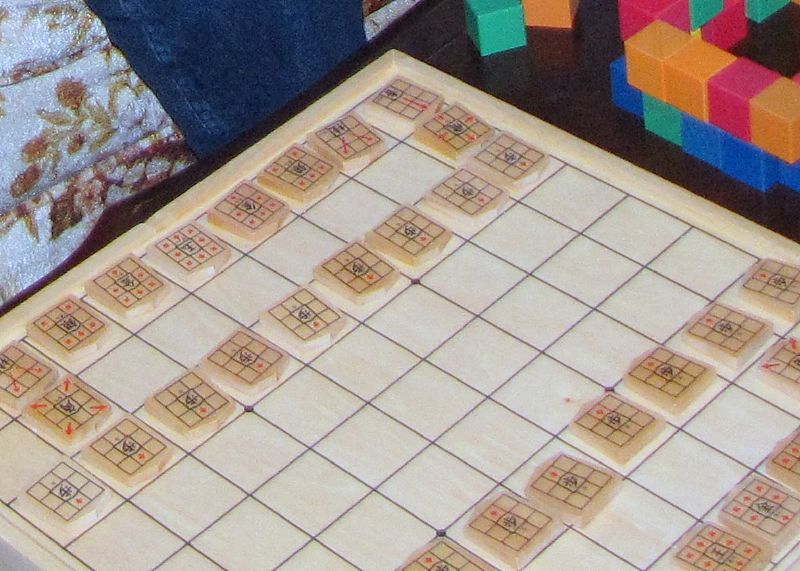This photograph showcases a complex board game set on a dark brown table. The game board is a white square grid made of thin black lines, forming an 8x8 layout. Each square contains a trapezoidal wooden playing piece, marked with a 3x3 grid of smaller squares. In the center of each piece, a distinctive Asian symbol is present, and various red arrows indicate possible moves. The scene is well-lit, highlighting intricate details like the red markings and the black squares.

To the left side, partially visible, is a flowery fabric piece, possibly a cushion or blanket, against what seems to be a floral-patterned sofa. To the right, scattered on the dark-colored floor, are small cubed building blocks in vibrant colors of orange, red, blue, and green. Additionally, a person in jeans, likely sitting on the floral sofa, is faintly visible, adding a touch of everyday life to the setting.